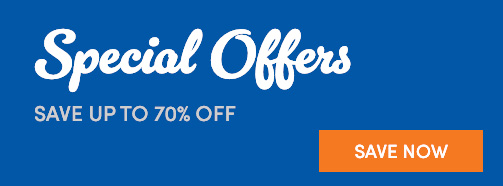The screenshot features a promotional banner set against a blue background. At the top, "Special Offers" is prominently displayed in white cursive-like lettering. Below this, in a slightly off-white gray font, the text "Save up to 70% off" is visible, standing out as the main message. In the bottom right corner, an eye-catching orange rectangle contains the call-to-action "Save Now" in white lettering. This orange button invites users to take advantage of the current deals. The design is straightforward and focused on drawing attention to the offer and the action button.